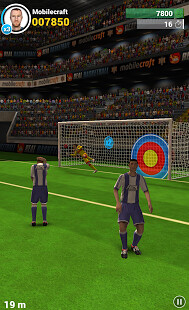The image appears to be a screenshot from a video game, likely a soccer simulation. The scene captures an action-packed moment on a vividly green soccer pitch. Two players, dressed in blue and white soccer uniforms, dominate the foreground, poised to make a play. Behind them, a detailed soccer net stretches across the frame, with a distinctive bullseye target to the right of the net. The bullseye features a white border, a blue outer circle, a red middle circle, and a prominent yellow center.

On the left side of the net stands the goalie, distinguishable by his gold uniform, ready to defend. A bright yellow line cuts across the lush green pitch, adding to the visual dynamism of the scene.

In the upper left corner of the image, the text "mobile craft" is displayed alongside a character resembling a white man, potentially a player or part of the game's graphics. Below this, a score of "007850" is prominently shown in gold lettering, adding to the competitive atmosphere of the game.